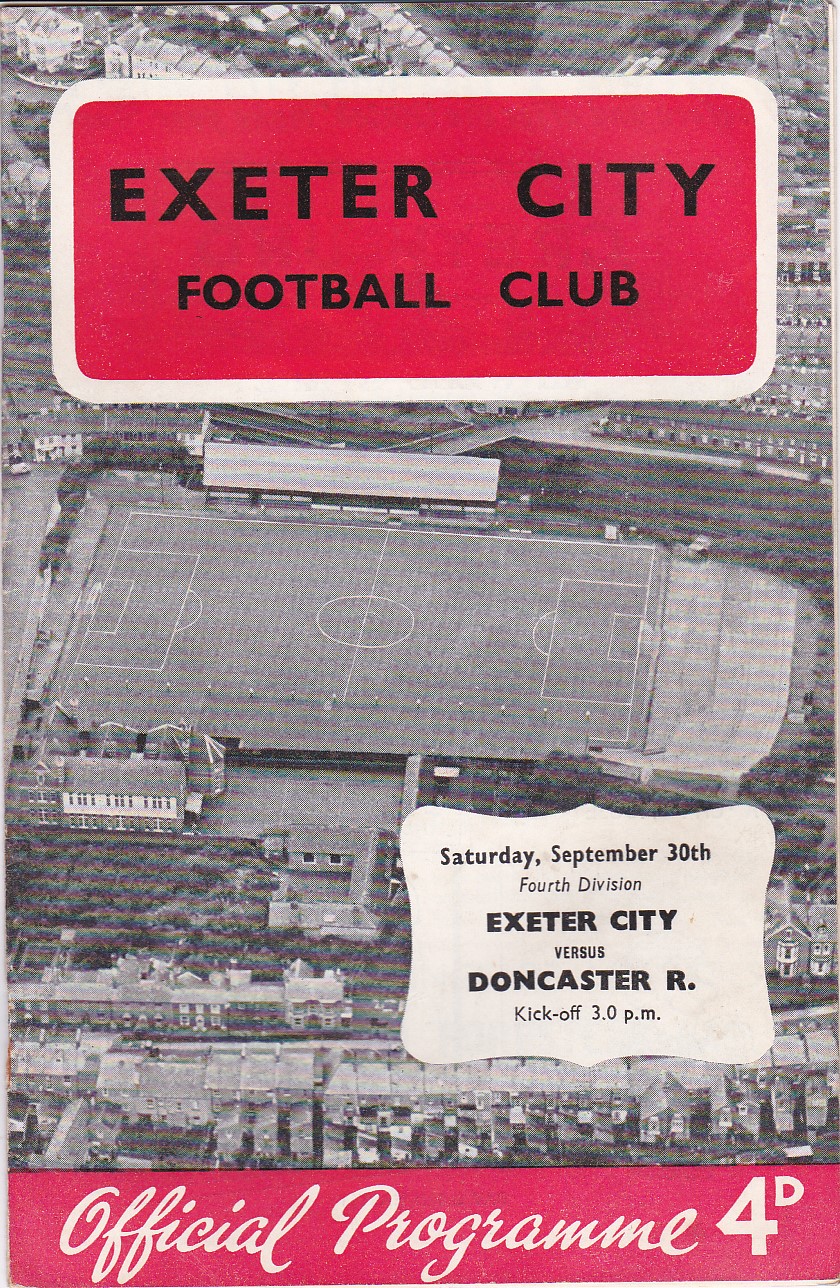The image features the cover of an old and slightly worn soccer program for Exeter City Football Club. At the top, a red banner outlined by a white line prominently displays "Exeter City Football Club" in bold black letters. Below this, a grainy black and white aerial photograph provides a bird's eye view of the stadium. In the lower right corner, a beveled bubble contains the text in black font: "Saturday, September 30th, 4th Division, Exeter City vs. Doncaster R, kickoff 3 p.m." At the very bottom, another red banner stretches across the width of the cover, featuring the cursive script "Official Program 4D" in white.